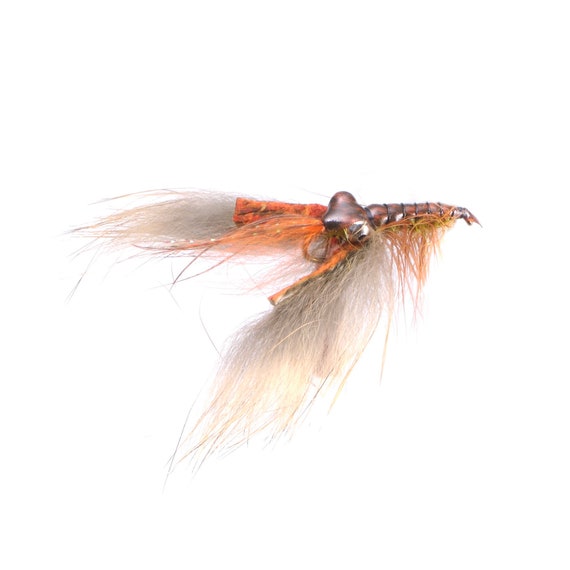This image showcases a detailed close-up of a fishing lure, set against a transparent background with a furry plume and a distinctive insect-like appearance. The lure features a metallic head that is a mix of silver and gold, with a body accented in gray, white, and orange hues. The head has an intricate design that somewhat resembles a fly, complete with large eyes on the sides.

Emanating from the body are long, hair-like extensions in gray and orange that give the illusion of antennae and segmented parts like a lobster's tail. Additional features include white feathers that fan outwards and are dark gray towards their base, turning stark white at the tips. Around the middle section, the lure appears to have a wire wrapping, adding to its intricate craftsmanship. This central wire extends downward, forming a heart shape, with multiple orange and yellow strings or feathers branching out beneath it, enhancing its visual complexity and mimicking the vibrant pattern of a bee.

The overall design is meticulously crafted to attract fish, utilizing a blend of lifelike insect characteristics and eye-catching colors, ensuring it stands out in its aquatic setting.